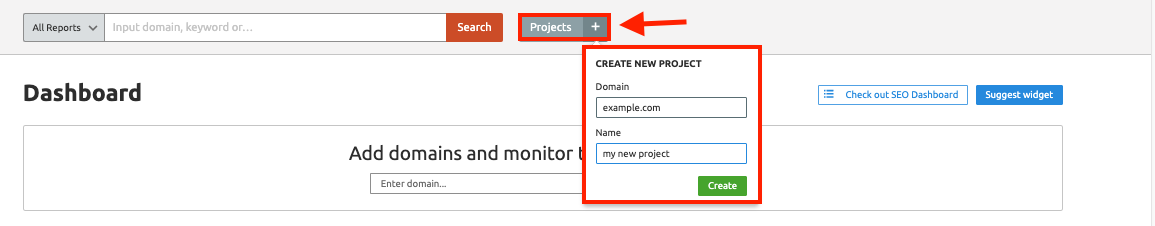A screenshot displays a website dashboard, which appears to be a domain tracking or monitoring tool. The user interface has a section labeled "Projects" prominently highlighted with a red box and arrow, alongside a plus sign. This suggests an actionable feature for creating a new project. A popup window partially obscures the phrase "Add domain to monitor," indicating a key functionality of the platform. The popup window is titled "Create New Project" and contains input fields for "domainexample.com" and a project name labeled "My New Project." This suggests that the user can enter a URL to initiate monitoring or tracking of a specific website, possibly to oversee its uptime, performance, or other metrics. The detailed elements combined hint at a robust platform designed for domain management and project creation.